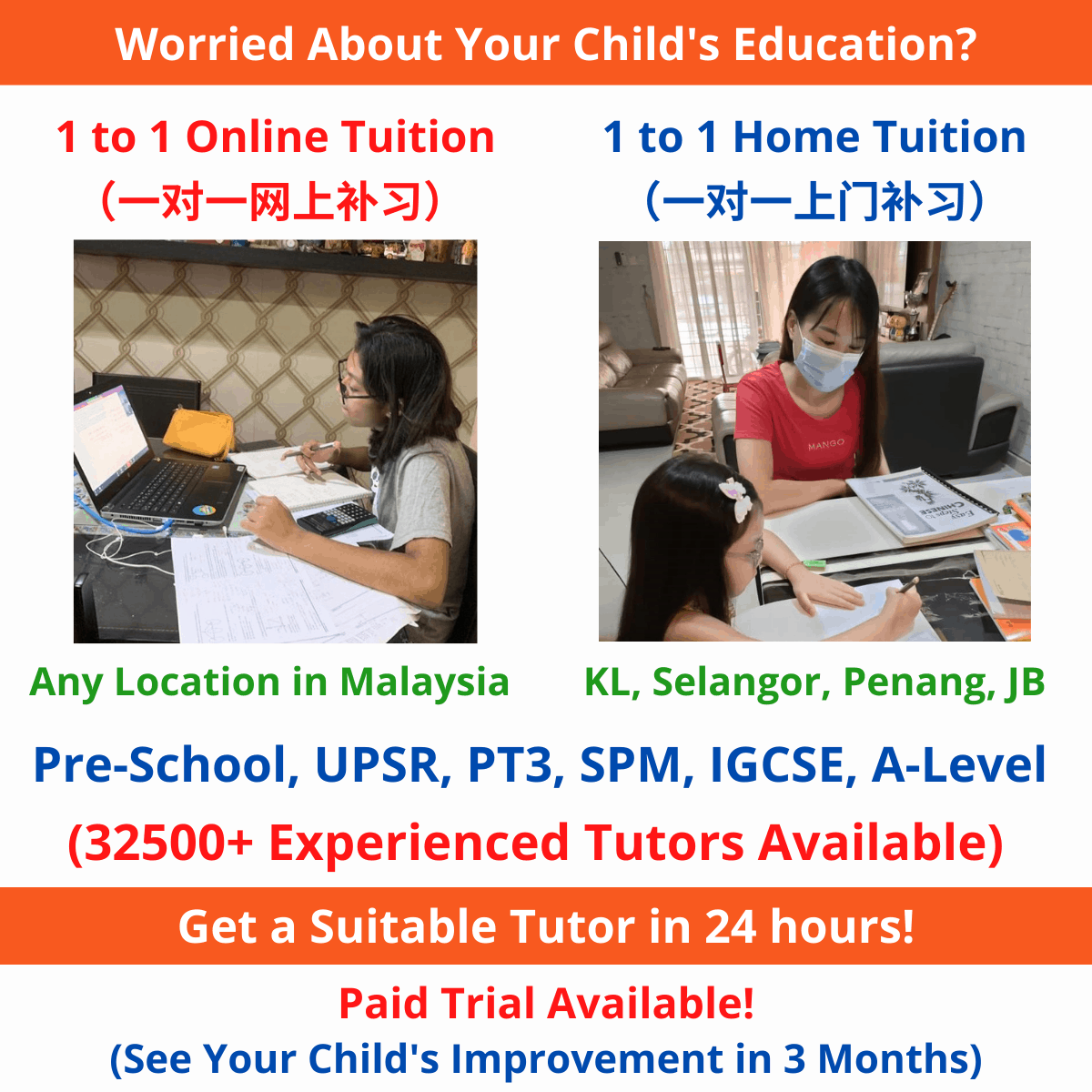This image is a colorful screenshot from an advertisement promoting a tutoring service. At the top, an orange bar features the question, "Worried about your child's education?" in bold text. Below, set against a white background, are two side-by-side images illustrating the service options. 

The image on the left highlights "One-on-One Online Tuition" available for any location in Malaysia. The adjacent image on the right emphasizes "One-to-One Home Tuition" specifically in Selangor and Penang. The advertisement boasts a network of over 30,000 experienced tutors ready to provide assistance.

Key features include: finding a suitable tutor within 24 hours, the availability of a paid trial, and a promise of noticeable improvement in your child's performance within three months.

The text is written in English along with a secondary language, likely an East Asian language, suggesting the tutoring service caters to a diverse clientele.